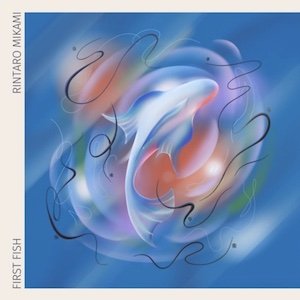The image appears to be a piece of abstract, contemporary artwork, potentially serving as album or book cover art. It prominently features the text "Rintaro Mikami" and "First Fish," suggesting that Rintaro Mikami is the artist and "First Fish" is the title. The central focus of the artwork is an abstract representation of a fish, possibly a koi or angelfish, set against a dynamic backdrop of swirling colors. The fish is depicted in shades of blue, white, red, green, and orange, with additional swirls of pinks, purples, and blacks creating a vibrant, effervescent atmosphere. The fish’s body curves gracefully, with its tail arching to one side and its fins downwards, giving it a flowing, almost ethereal quality. The backdrop includes a blend of rounded, multicolored swirls that add to the abstract, modern aesthetic of the piece. The overall composition is intricate and allows for varied interpretations, inviting the viewer to immerse themselves in its contemporary, imaginative design.